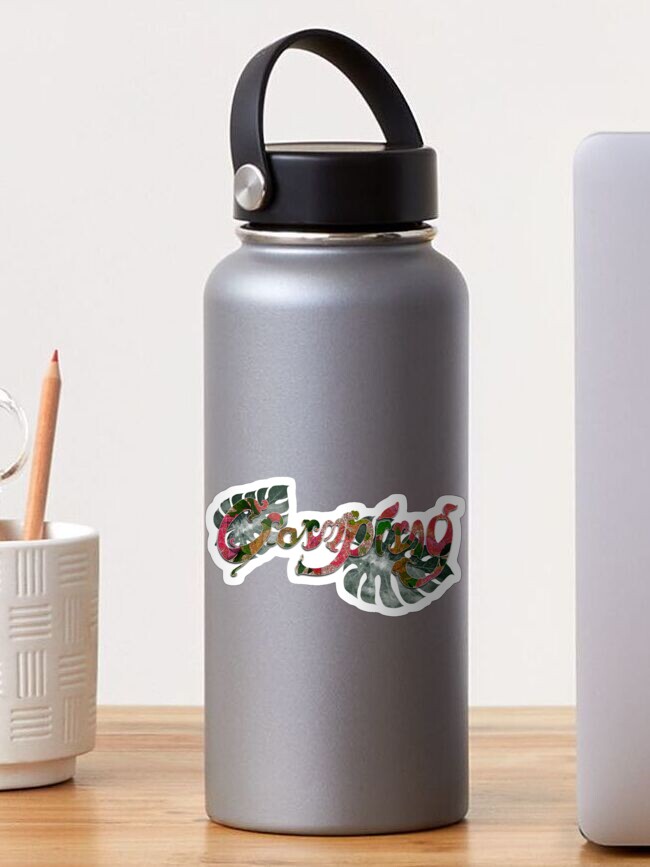The image showcases a detailed scene centered around a bottle, prominently placed on a wooden table. The bottle features a sleek, silver-grey metal body with a black plastic top. A colorful sticker decorates its midsection, displaying green leaves and partially visible text that includes "CO." To the bottle's left sits a white ceramic mug containing a pencil with an orange tip and a pair of scissors. On the right, part of a laptop is visible, contributing to the organized yet lived-in ambiance of the scene. The background wall is a soft grey, enhancing the visual calmness and emphasis on the items on the table.